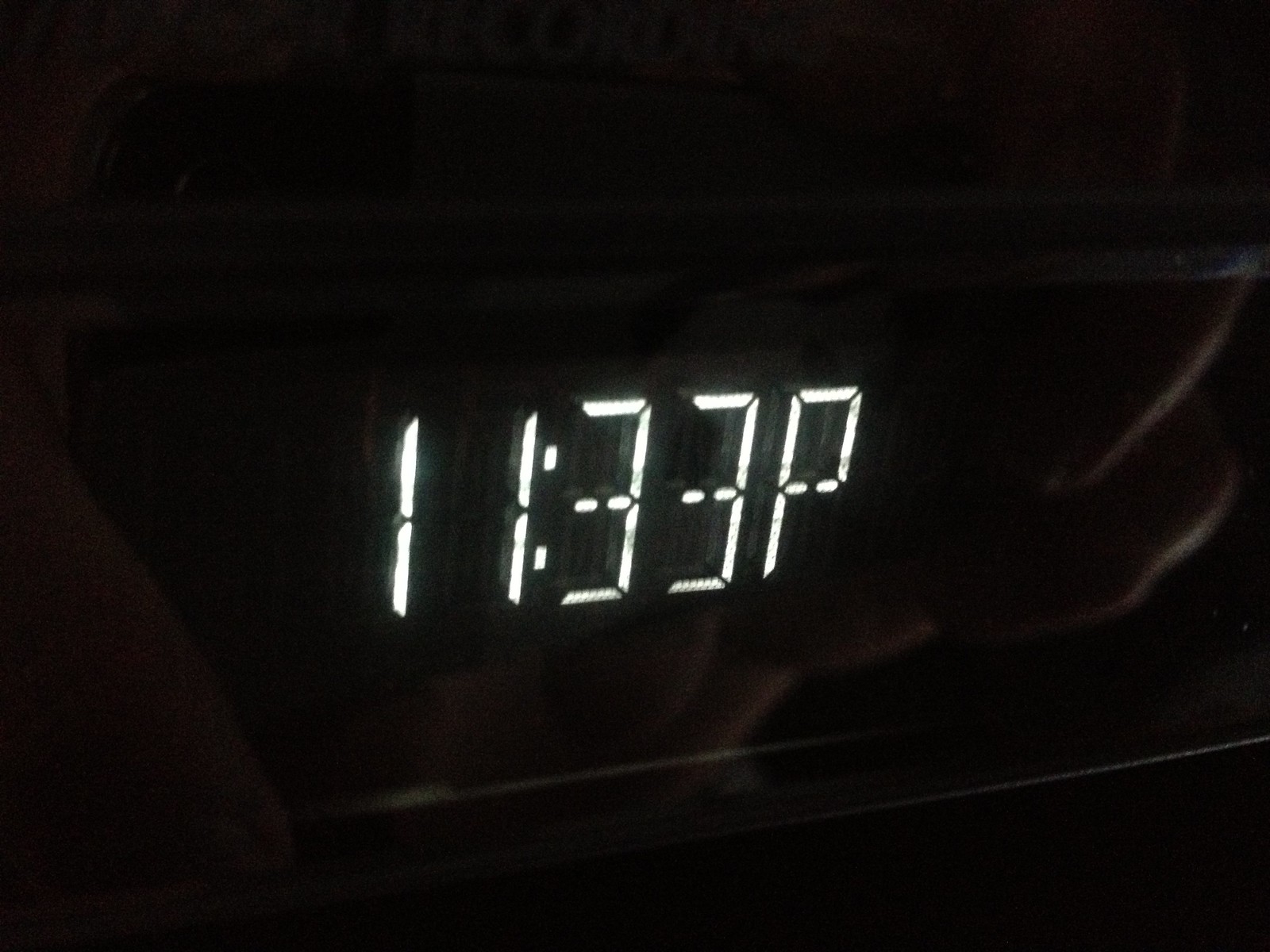The image captures a dimly-lit kitchen enveloped in darkness. At the center, a digital clock emits a faint glow, displaying the time "11:33 PM" in bright white numerals. The rest of the scene is shrouded in obscurity, with only vague, indistinguishable reflections hinting at the surrounding appliances and surfaces. The stark contrast between the luminous clock display and the otherwise pitch-black environment creates an eerie, almost solitary atmosphere.